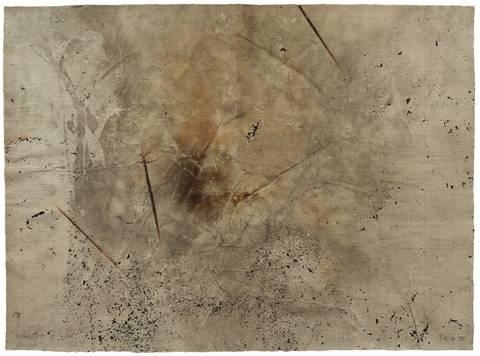The image portrays a highly abstract and aged piece of what appears to be print or an old, neglected paint board. Dominated by a palette of grays, blacks, and browns, the image features a central brown spot that is encircled by varying shades of gray, creating a layered effect. Over the brown spot, there is an indeterminate figure or scribble, adding to the image's mystery. The surface is marred with black lines, dots, and paint splashes, as if the material—perhaps a wrinkled, ironed-out piece of paper or canvas—has endured significant wear and tear. The background, resembling a discolored and aged tan, further contributes to its weather-beaten appearance. Overall, the image gives an impression of something that has been left to time, showing numerous wrinkles, cracks, and discolorations without any discernible shapes or objects, making it a perplexing, yet intriguing, visual.